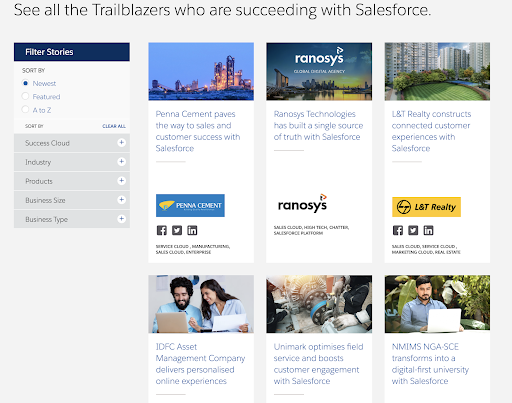**Caption: Trailblazers Achieving Success with Salesforce**

At the top of the page, the headline reads, "See All the Trailblazers," highlighting the pioneering individuals and companies excelling with Salesforce.

To the left, a filter section allows users to sort stories, with options including:
- **Newest:** Indicated by a blue dot
- **Featured:** Indicated by a white dot
- **A to Z:** Indicated by a white dot

On the right, showcasing a series of success stories:

1. **Pena Cement:** Features a cityscape at night, with tall buildings and lit-up windows. The caption reads, "Pena Cement paves the way to sales and customer success with Salesforce."
2. **Raynos Technologies:** Displays another nighttime city scene by the water, stating, "Raynos Technologies has built a single source of trust with Salesforce."
3. **L and T Realty:** Depicts more tall gray buildings, captioned, "L and T Realty constructs connected customer experiences with Salesforce."

On the bottom row, left to right:

1. **IDFC Asset Management Company:** Shows two people with black hair smiling in front of a computer. The caption says, "IDFC Asset Management Company delivers personalized online experiences."
2. **Final Square:** Features a man with black hair and a black beard sitting in front of a laptop, with plants in the background.